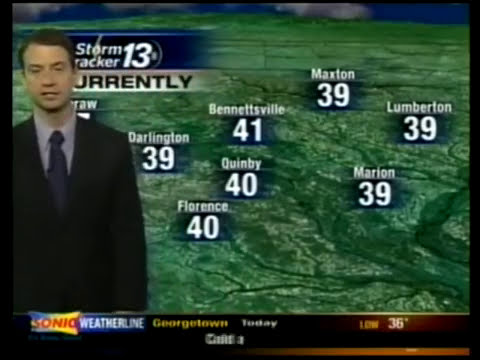The image is a slightly blurry, VHS-quality screenshot of an older weather report broadcast. On the left side of the image stands a young male weather reporter. He has short brown hair and is dressed in a black suit, blue tie, and light-colored shirt. The top left corner of the screen displays the "Storm Tracker 13" logo, indicating it's a current temperature update. In the background, a green map shows topographical features and temperatures for various cities, including Marion, Lumberton, Florence, Darlington, Bennettsville, Maxton, and Quimby, with readings around 39-41 degrees. A horizontal banner at the bottom reads "Sonic Weatherline Georgetown Today" and indicates a low of 36 degrees for Georgetown. The banner also features a yellow and red Sonic restaurant logo, marking the sponsorship of the weather segment. The overall image captures the essence of a vintage weather forecast with the essential details prominently displayed.